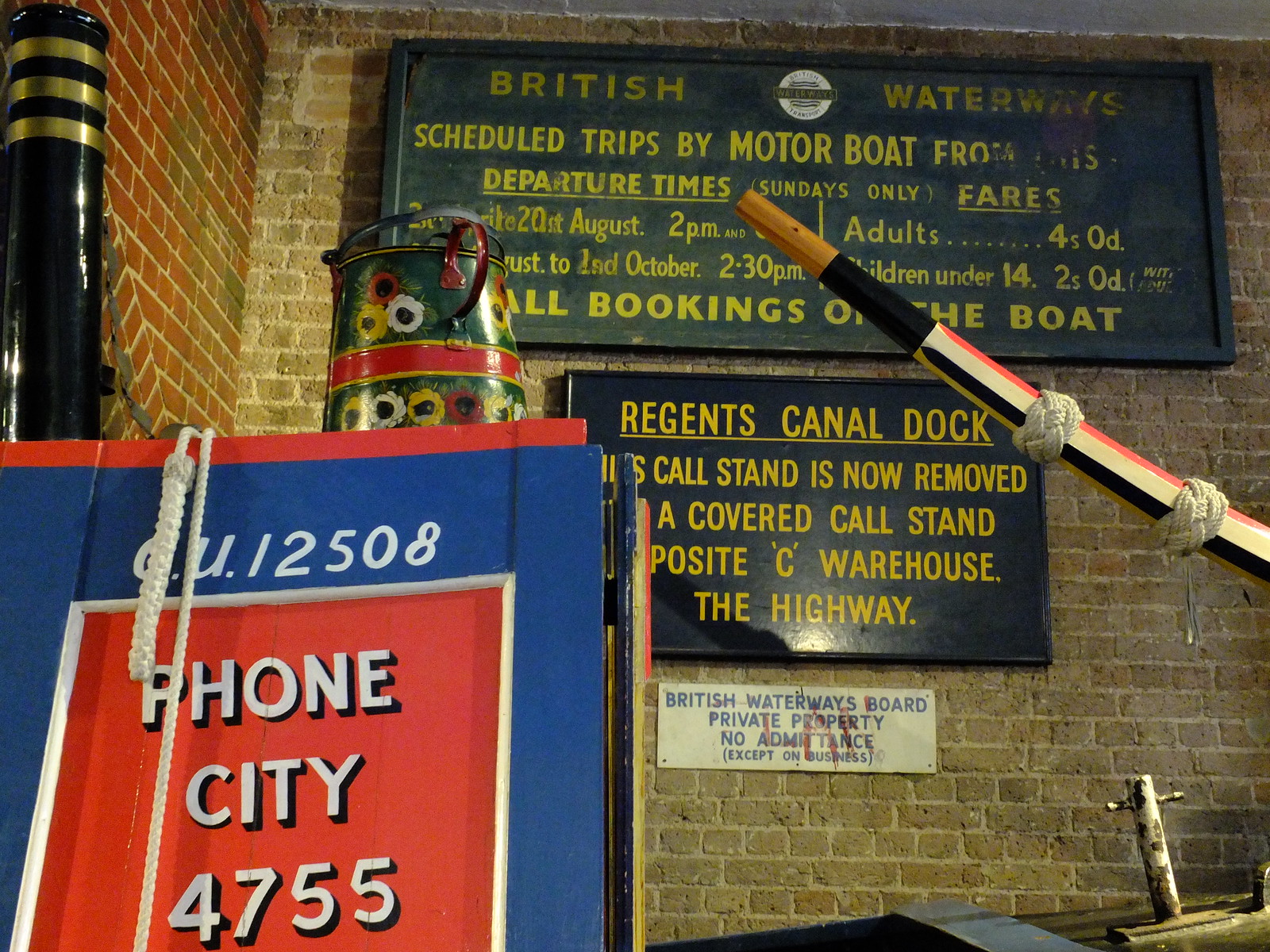This image captures a collection of various signs affixed to an old, tall wall made of light gray and red bricks with some additional free-standing elements. Dominating the top of the wall is a large, dark green sign with gold letters that reads "British Waterways". It details scheduled motorboat trips, with specific times and fares listed for adults and children. Directly beneath this is a black sign, also with gold letters, which states "Regents Canal Dock" and provides further information about the dock, such as the removal of the call stand. Below this black sign, there is a small white plaque with the inscription "British Waterways Board, Private Property, No Admittance" accompanied by some red graffiti markings. To the bottom left of the image, there is another notable sign: a blue one featuring a red interior and white lettering that says "Phone City 4755". Additionally, a tin pail with painted flowers and a red border sits atop a freestanding element next to the signs. The scene is completed with an oar crossing diagonally from the center right up into the green informational board at the top, and a white rope hanging off the blue "Phone City 4755" sign.